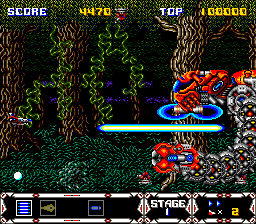The image is a small, pixelated screenshot from a very old video game. Dominating the right side of the image is a robotic-like creature with a bright red and silver body. The robot has a distinguishing bright blue visor and is emitting a bright blue infinity sign from its mouth. It features a long arm constructed from interlinked metal circles, ending in a large red claw with metal points at its tip. The robot is depicted as shooting a blue and yellow laser beam. Accompanying the robot are two small floating ships, one situated on the left side and another directly below it.

The backdrop of the scene is divided into two main color sections, with a green bottom and a lighter green top, sporadically decorated with trees. At the top of the image, "SCORE" is displayed in white lettering outlined in blue. Below this, the score "4470" is highlighted in yellow. Adjacent to the score, the word "TOP" is present in the same blue-outlined white font, and the number "100000" appears in yellow print beside it. The bottom of the image features a platform on which the robotic creature is positioned. Additionally, texts indicating "stage one" and the number "two" are displayed in this area.